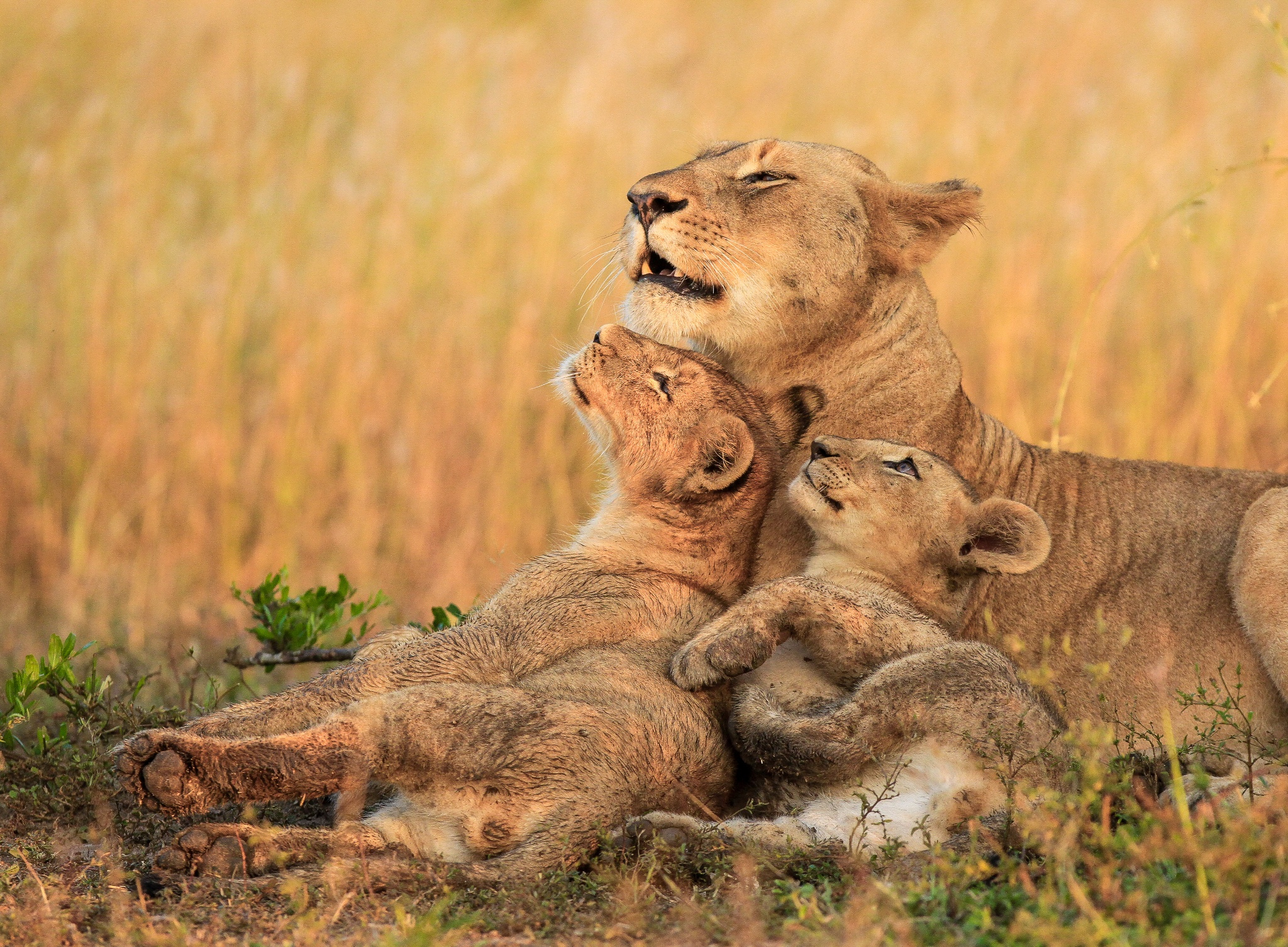The photograph captures a serene moment of a lioness and her two cubs resting together in a sunlit grassy field. The dry, light tan grass in the background is slightly blurred, bringing focus to the central figures. The lioness, with her eyes closed and mouth partially open, is lying on the ground with her cubs close by. The cubs, one appearing older and possibly male, and another smaller one, nuzzle affectionately under their mother's chin, both looking up at her. The family’s fur ranges from light brown to almond, accentuated by black noses and eyes. Scattered throughout the field are patches of green vegetation, including a tree branch with a few green leaves near the ground and some green weeds in the bottom right corner. The overall atmosphere reflects a peaceful, daytime scene in a light brown grassland, emphasizing the close bond of the lioness with her young cubs.